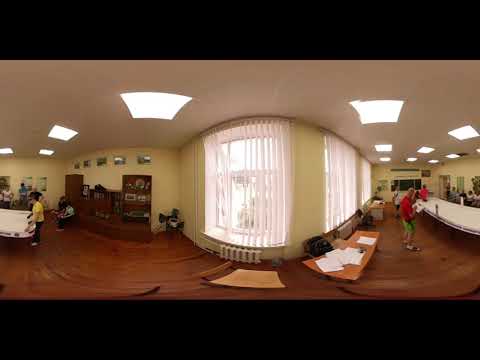The image captures the interior of a community center characterized by a light greenish-colored wall and a white ceiling fitted with lights. The floor is made of wood paneling. Central to the image is a window with white vertical blinds partially open, revealing a sunny day outside. People are congregated on both sides of the room, and some are standing while others are sitting.

On the left side of the image, there's a group of people near wooden furniture adorned with books and photographs. Among the visible details, there's a person in the foreground on the right side wearing a red top and shorts, and another person in the background also dressed in red. A white countertop is positioned in this area, accompanied by a wooden tabletop below, scattered with white papers. The right side also features a larger white table where more people are gathered.

In the left center of the image, a wooden bookshelf displays various framed items and objects. Further to the left, possibly a foosball or shuffleboard table can be identified amidst the gathering of people. Overall, the setting conveys a lively community space filled with interaction and casual activities.